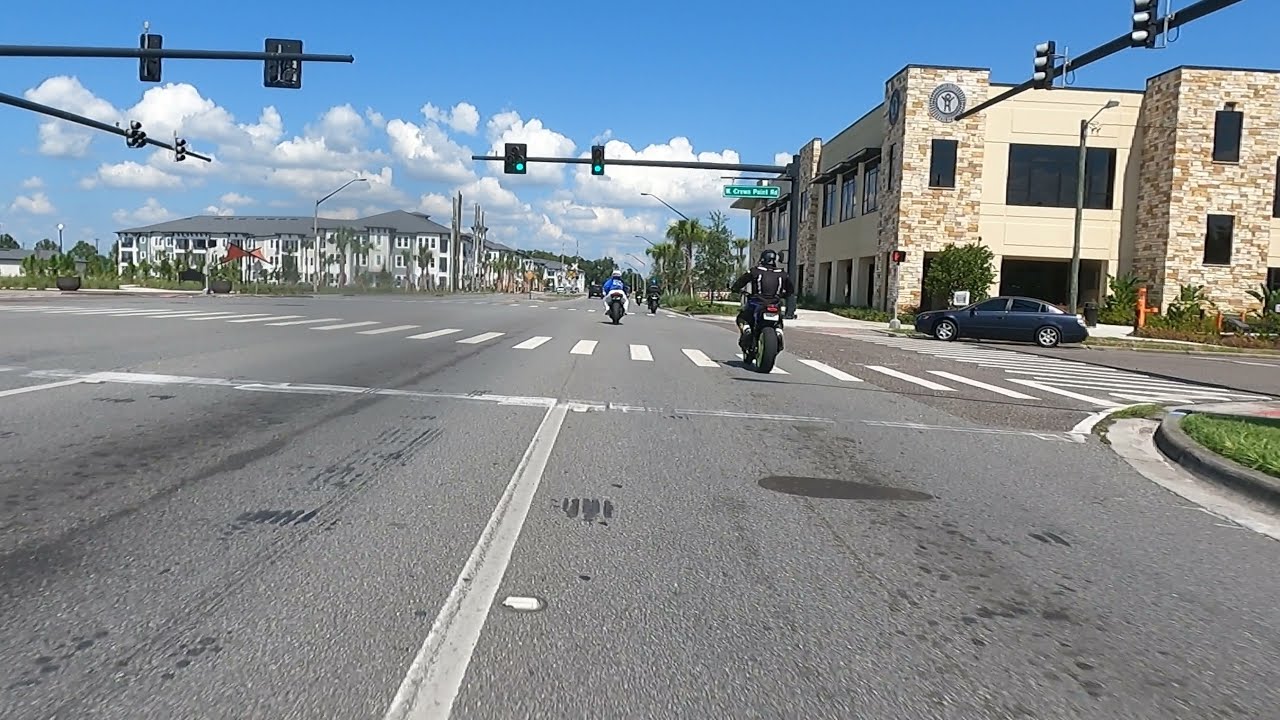The photo captures a vibrant, daytime scene at a bustling four-way intersection with a crosswalk. Multiple motorcycles, at least two visible and possibly more in the distance, are riding through a green light. To the right, a blue Nissan Altima is preparing to make a right turn. Surrounding the intersection are various buildings, including a two-story white building with brick columns on the left corner and a tall, white apartment complex in the far upper left. There is a mix of other multi-story buildings, including a brown brick building on the right and a gray and white structure nearby. A green street sign reads "Creek Road," indicating the location. The scene is framed by a clear blue sky adorned with occasional white, fluffy clouds. Traffic lights are positioned at all four corners of the intersection, ensuring orderly movement of vehicles and pedestrians. Sidewalks with stretches of grass line the streets, and a distinctive building on the right with a blue circle emblem featuring a human figure adds to the area's character.